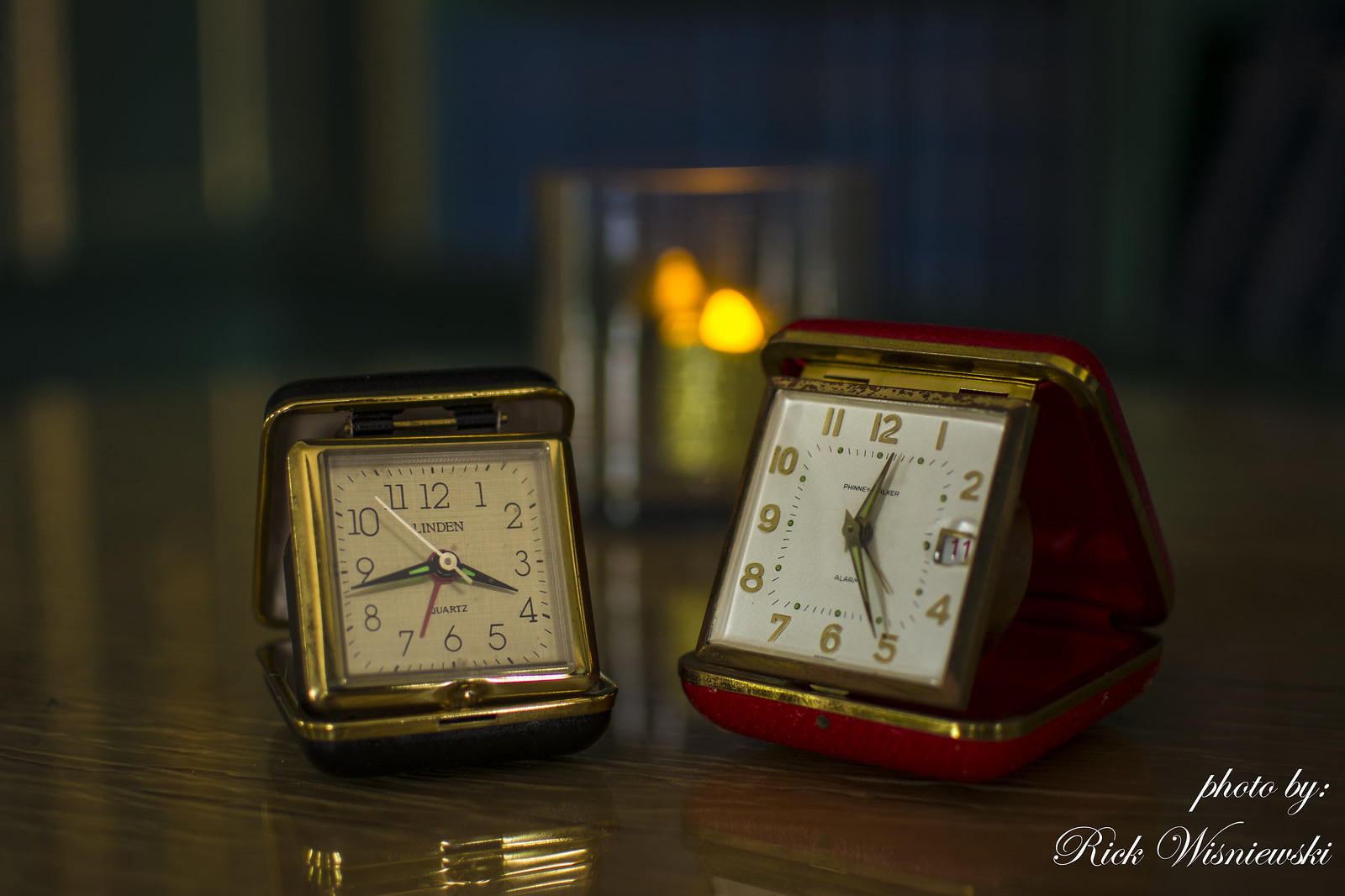The image shows two collapsible travel table clocks, reminiscent of those used in the past. Both clocks have square faces and are positioned facing each other on a shiny brown table. The background transitions from a brown section with three light brown vertical stripes on the left to a blue area on the right, possibly resembling a window. 

The smaller clock on the left features a gold face with a high-polished yellow gold border, black hands with fluorescent green lines near the center, and the name "Linden" on the face. Its black casing has gold trim, and the off-white face is adorned with black numbers.

The larger clock on the right has a red casing with gold trim. Its face is gold-tinted with gold numbers and hands, and a white background. Instead of the number three, there is a small square cutout displaying the day of the week with an '11' visible. Unlike the smaller clock, this one does not have a second hand.

In the bottom right corner of the image, the text "photo by Rick Wisniewski" can be seen. Behind the clocks, there is a blurred object resembling a glass with a green candle and two small flames.